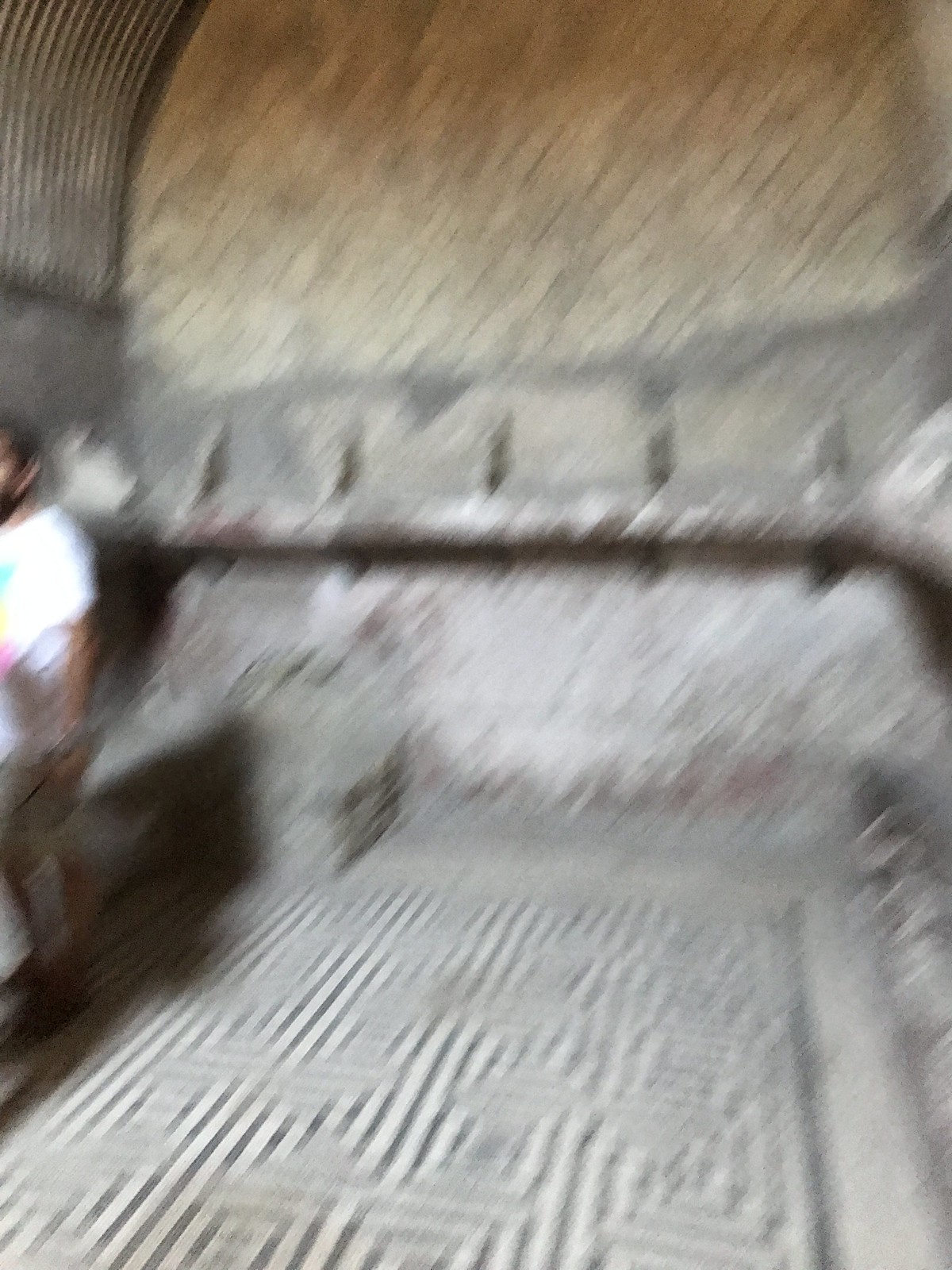This blurred indoor photograph captures an unearthed Roman ruin that exudes architectural and historical significance. The focal point is the mosaic floor adorned with geometric, maze-like patterns composed of black lines that create intricate interlocking rectangles, although the details are obscured by the blur. The floor is uneven, hinting at different depths throughout the room. Surrounding this central feature, the plaster walls exhibit a mix of reddish, white, and gray tones, with uneven patches that jut out, indicating wear and age. The left side of the image shows an arching ceiling transitioning from a light beige to a darker brown at its apex, highlighting its historic construction. There are individual bricks and stones visible in parts of the wall, some appearing ribbed and engraved, suggesting once-painted surfaces now marred by time. A person with olive skin, short black hair, and a short beard, dressed in a white t-shirt with cyan, yellow, and pink accents and tan khakis, stands near the background but is partially cut off. Overall, the image captures a dimly lit, damp environment that might be a cave or basement-like setting, adding an air of mystery and antiquity to the scene.